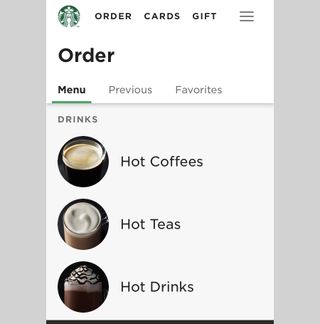This image appears to be a screenshot from the Starbucks app. The main background of the page is a light gray or light purplish-gray, with a smaller rectangular vertical box overlaying it. The top third of this vertical box features a white background, while the remaining portion is light gray.

In the upper left corner of the white background, the iconic Starbucks logo is displayed within a circle. To the right of the logo, bold black text reads "Order Cards & Gift." On the far right, three horizontal lines symbolize a menu for additional options.

Below this header, larger bold black text prominently labels the section as "Order." Directly underneath, there are three navigation options: "Menu," "Previous," and "Favorites" in light gray text. However, the "Menu" option stands out in black text with a green underline, indicating it is currently selected.

The rest of the screen shifts to a light blue background. At the top, the word "Drinks" appears in dark gray text. Beneath this heading, three categories are listed in dark gray text: "Hot Coffees," "Hot Teas," and "Hot Drinks," each accompanied by a corresponding image of a drink.

At the bottom of the vertical box, a thin black ribbon spans the width of the screen. This design element adds a finishing touch to the clean and organized layout of the Starbucks app interface.